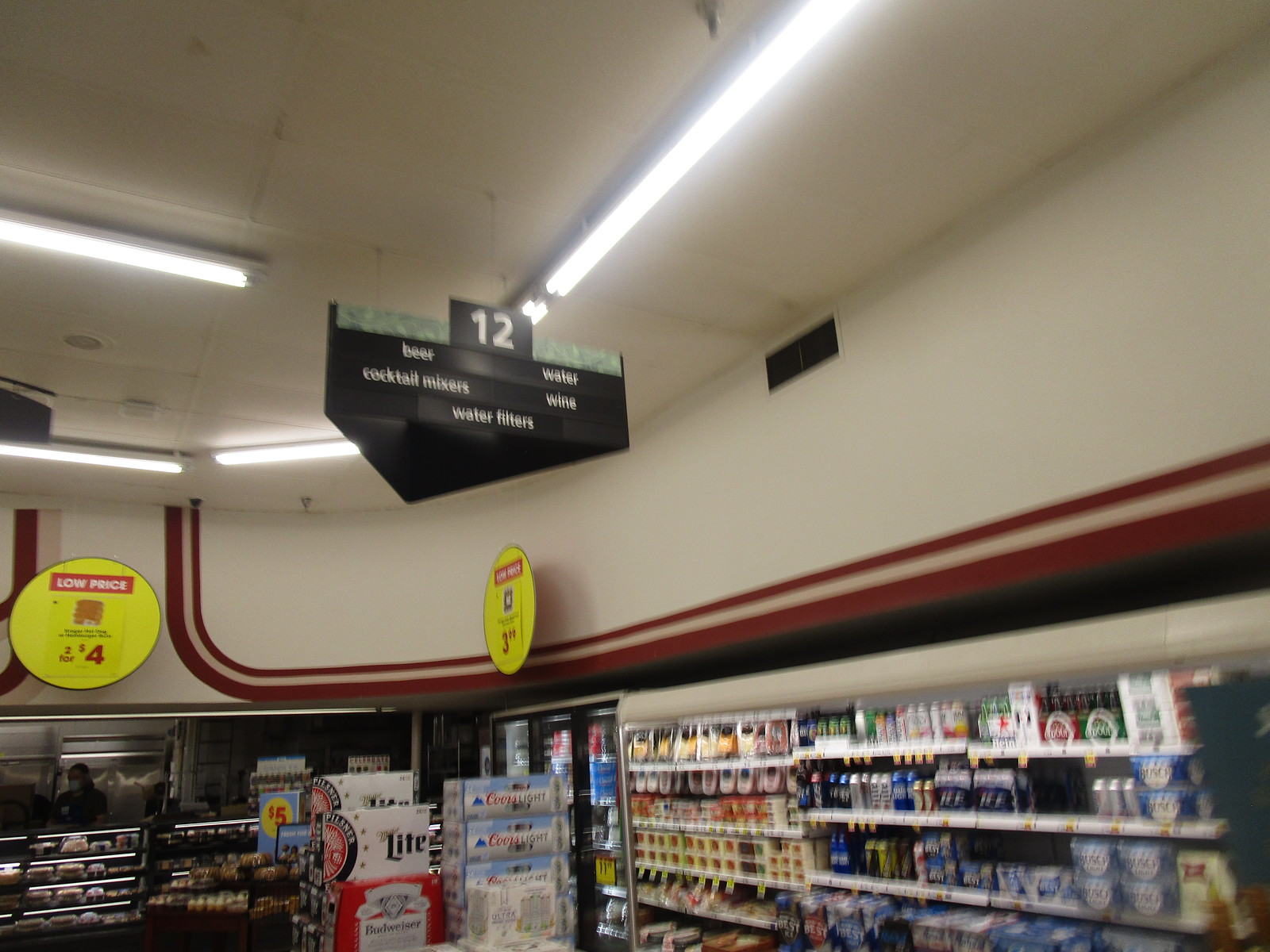In this photograph taken inside a grocery store, we see the alcoholic beverage and beer aisle situated in the corner of the store. The right side of the image is lined with a variety of beers for sale, showcasing a myriad of colors and brands. The photograph is slightly blurry, indicating it was taken quickly or without stabilization. On the left side of the image, there are cases of Coors Light and Miller Light beer stacked on top of each other, leading up to a refrigerated section behind them. Above this section are several signs, including a three-dimensional triangular sign highlighting the sections: beer, cocktail mixers, water, wine, and water fillers, marked with a white number 12. The overall atmosphere of the image conveys a typical, well-stocked grocery store's beverage corner.